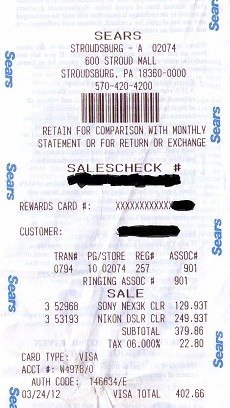A detailed caption for the image could read:

"A receipt from Sears located in Stroudsburg, Pennsylvania at the Stroud Mall (Store #02074, 600 Stroud Mall, Stroudsburg, PA 18360). The receipt includes a barcode and several important details. The receipt header indicates it is retained for comparison with monthly statements or for returns/exchanges. 

The Sales Check Number is prominently crossed out with black ink or marker, and the Rewards Card Number is partially inked out for privacy. The transaction was processed by store associate numbered 0794, with the regular association listed as 02074 and Ring Association Number 901. 

The sale included two main items: a Sony product listed as 'Next Clear' priced at $129.33 (taxable), and a Nikon DSLR on clearance priced at $249.93, bringing the subtotal to $279.86. With a sales tax of 6%, the tax totaled $22.80. 

The payment was made using a Visa card (card type listed as 'Visa Account W498B') with authorization code 146634E. The total amount paid on 03-24-12 was $402.66."